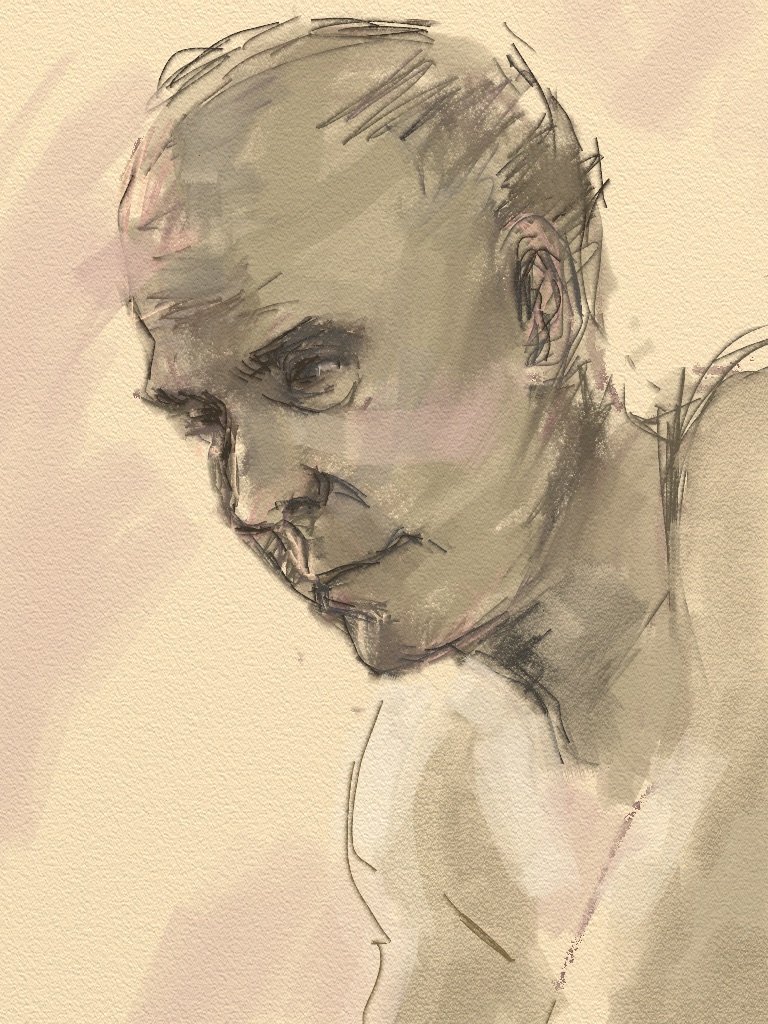This detailed illustration appears to be a pencil and possibly watercolor sketch of an elderly or middle-aged bald man, viewed in profile facing towards the left. The drawing, executed on a piece of textured paper, features advanced shading, particularly around the man's head, which is bald on top with wisps of hair on the sides. He has thick eyebrows, and a clean-shaven face with an intent expression and a slight smile. The man’s head is slightly tilted downward, suggesting a contemplative or bowing posture. Visible in the image are his left ear, part of his left shoulder, and his right shoulder, with the rest of his body extending out of frame. The background is predominantly white with occasional purple smudges, giving a dusty rose impression, enhancing the depth and contrast of the sketch. The image is vertically oriented, emphasizing the man's head and upper torso, with no photographic elements or writing present.